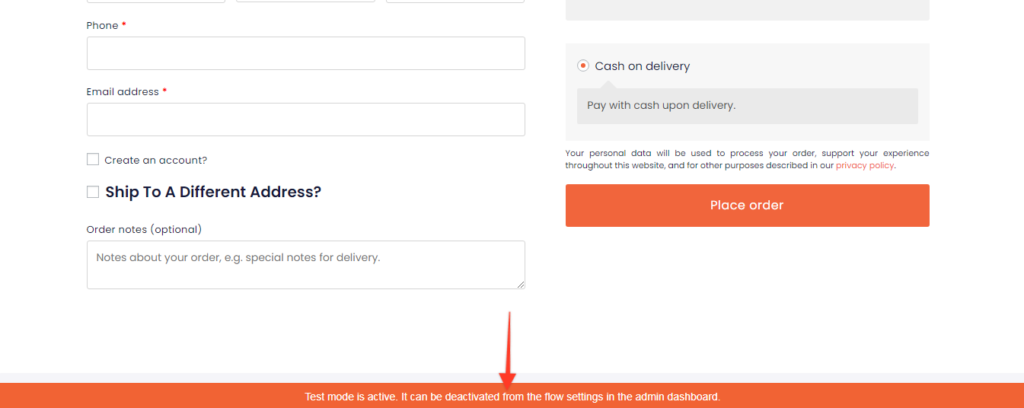In this image, a website's checkout system is depicted. At the very top left, there are input fields, though some portions are cut off. The visible sections include a field labeled "Phone" in black text, accompanied by a red asterisk to indicate it's a required field. Below this, there is an empty rectangular input box with a white background.

Next, the label "Email Address" appears, also in black and followed by a red asterisk. Similarly, an empty rectangular input box is situated below this label. 

Further down, towards the middle left of the image, there is a small checkbox next to the text "Create an account?" in black. Directly below this checkbox, there is another labeled "Ship to a different address?" in darker, bold black text.

Below these checkboxes, the text "Order Notes (Optional)" is visible, with a larger empty rectangular input box beneath it for additional information.

On the middle right side of the image, there is a prominent "Place Order" button, featuring white text on an orange background, indicating the final step to process the order.